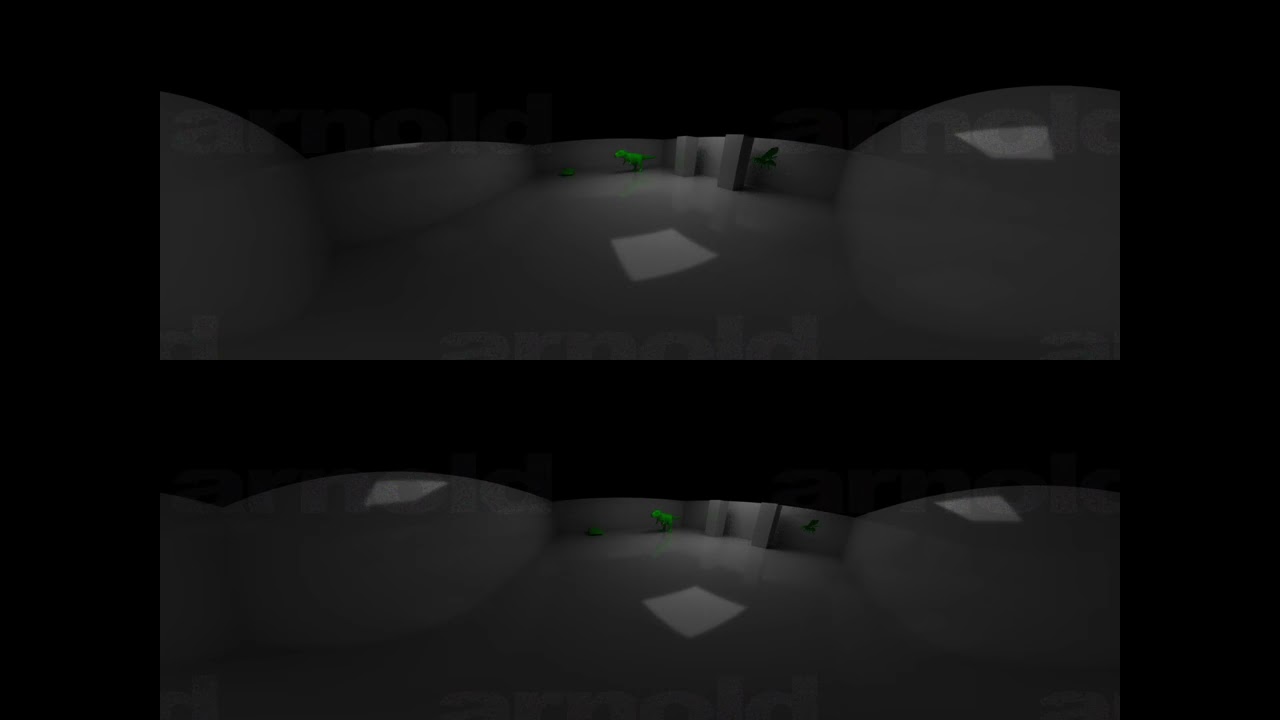This image showcases two nearly identical gray-toned computer-generated scenes placed side by side on a black background, separated by a thick black line. Each scene features a central white square on the floor, with two additional white squares on the walls arranged in a geometric pattern. There are notable green objects in the background: a larger one near the back wall and a smaller one positioned slightly away in the corner, both illuminated by a light source. The name "Arnold" is faintly visible at the bottom of each scene, though partially cut off. The overall dark tones and unclear details give the image an almost surveillance footage-like quality.